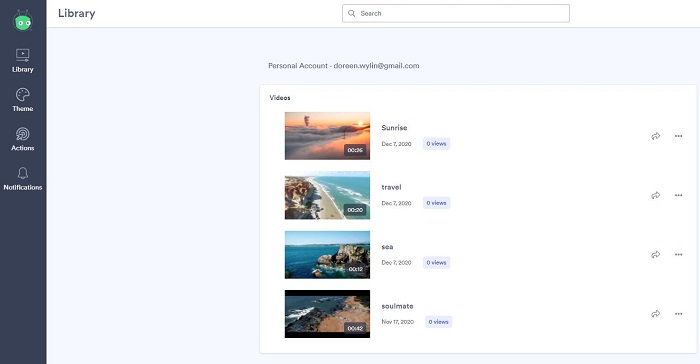The screen displays a library application interface. On the left, there's a vertical grey menu bar featuring several icons and labels: 

1. A green alien icon with white eyes and antennae, labeled "Library."
2. Below that, a painter's palette icon labeled "Theme."
3. Next, a bullseye with an arrow labeled "Actions."
4. At the bottom, a bell icon labeled "Notifications."

To the right of the menu bar, the top section of the page has a white background header with "Library" written in black. Adjacent to this, there's a search box.

The main body of the page is light grey. Prominently positioned at the top center, it reads "Personal account of Doreen.Wyland@gmail.com." Beneath this, there's a white box titled "Videos" that lists four videos. Each video listing comprises several columns:

- The first column contains a thumbnail image.
- The second column names the video.
- The third column shows the upload date.
- The fourth column features a small grey box displaying the number of views, with all videos currently showing zero views.
- The final column on the far right includes an arrow icon for accessing an additional menu, indicated by three horizontal dots.

Overall, the interface is user-friendly and organized for easy navigation and content management.